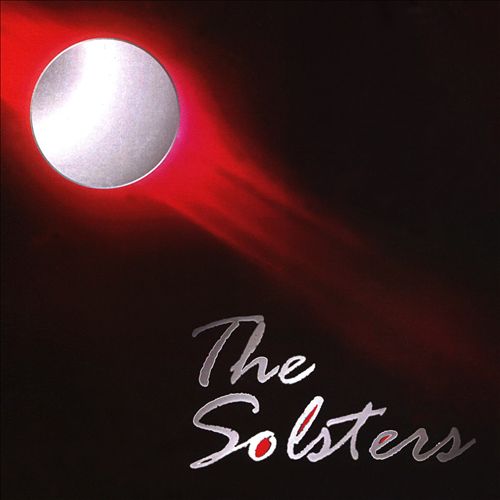The image appears to be a square-format cover, possibly for an album or book, featuring a minimalist and modern graphic design. Dominating the top left corner is a digitally rendered, silver circle that represents the moon, radiating a red glow with a streak extending diagonally towards the center, where it fans out into radial beams. The background is predominantly black, enhancing the contrast and visual impact of the elements. In the bottom right corner, elegant cursive script spells out "The Solstice" across two left-justified lines, with “The” on the top line and “Solstice” on the bottom. The script is primarily silver with portions of the letters 'O', 'L', and 'E' filled in with red, adding subtle color accents. The text features a slight gray shadowing to give it depth. This cover art brilliantly combines color illustration and typography to create a striking visual effect.